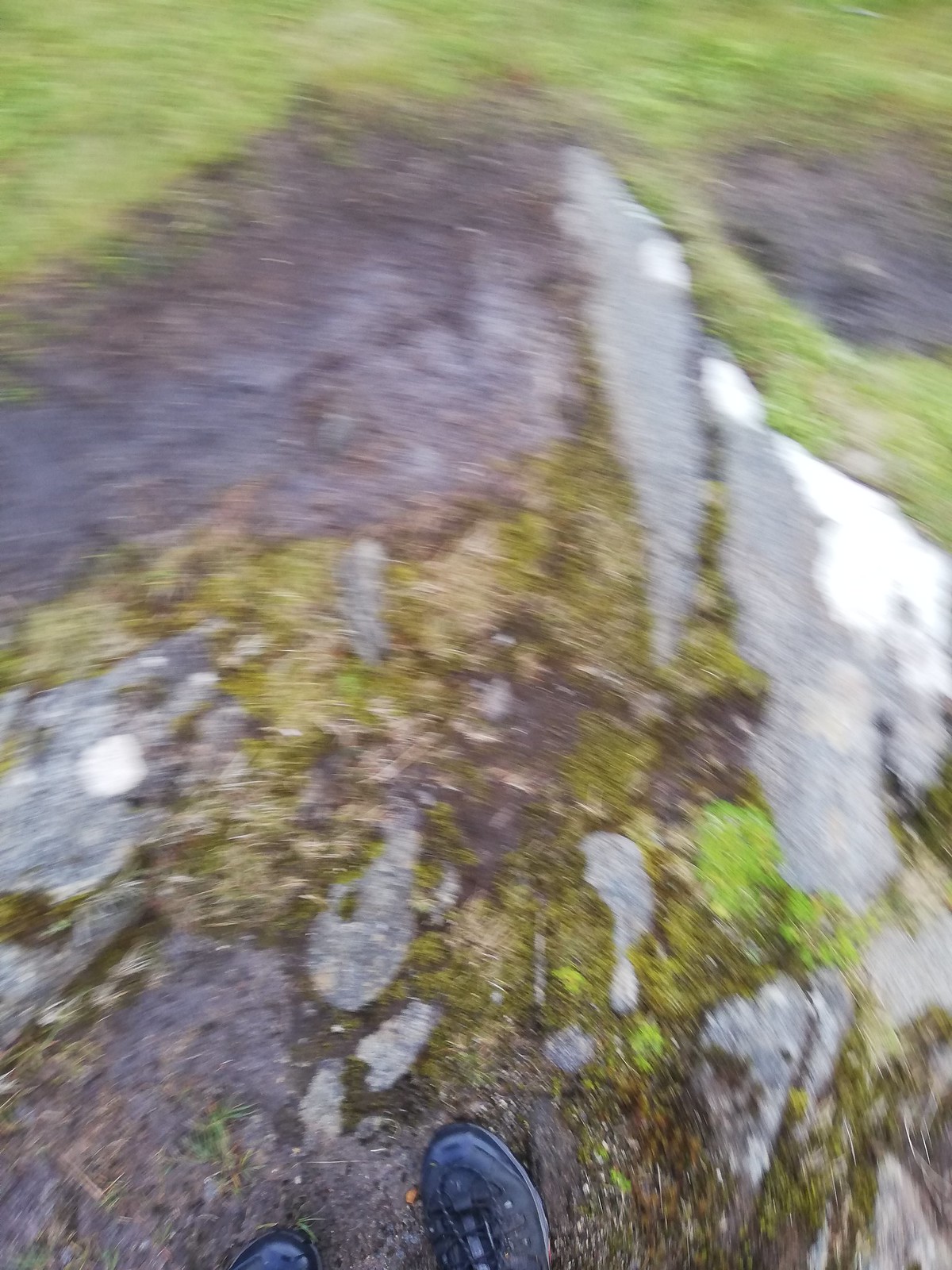This photograph appears to be taken from an action camera worn by someone standing still or in slight motion on a rocky terrain. The perspective is looking downward, capturing the person's feet clad in black, or possibly bluish, lace-up shoes, clearly visible at the bottom edge of the image. The surrounding area features large rock outcroppings, with the rock surfaces being partially obscured by thick moss and lichen, contributing to a richly variegated texture. The colors range from light and dark green of the moss, interspersed with gray and brown rock surfaces, with some areas of white that could be either light reflections or lichen. The overall image has a slightly blurred, abstract quality reminiscent of a Van Gogh painting. The upper portion of the image reveals green grass, suggesting the presence of more ground vegetation beyond the immediate rocky foreground.